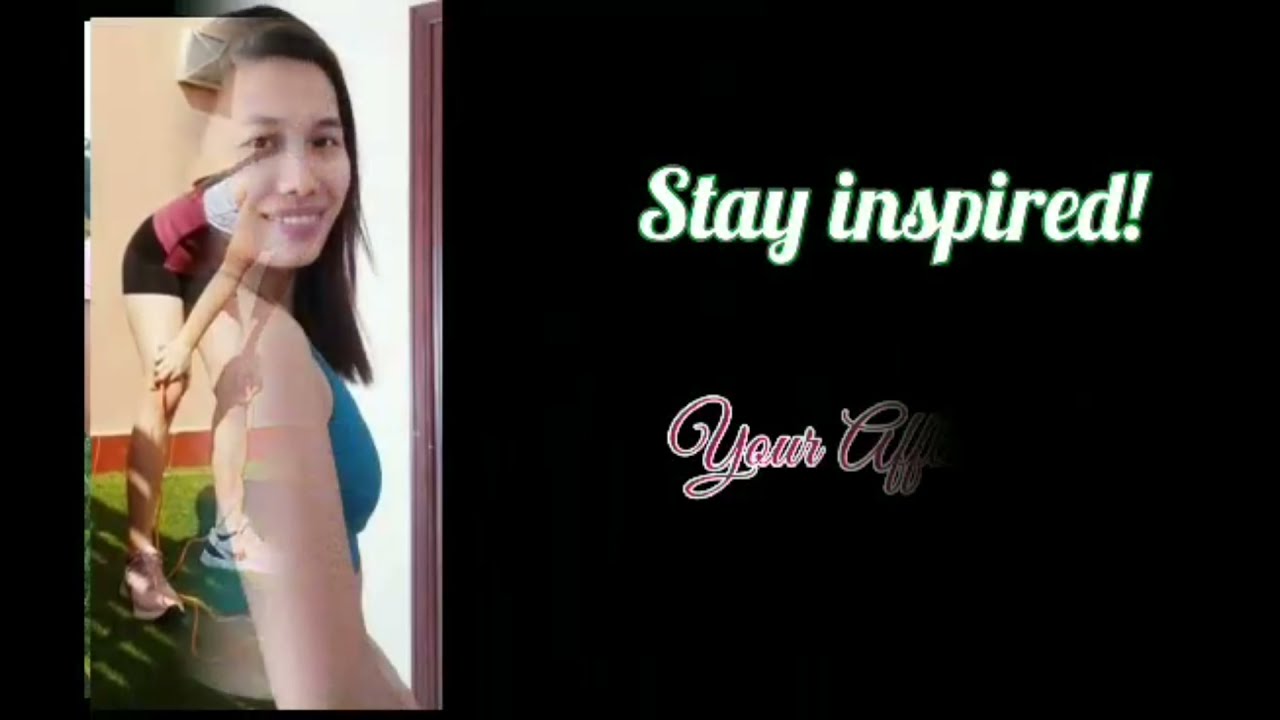The image features a multi-layered, semi-translucent composition on a completely black background. On the left side, there's a blended depiction of two women. The first woman, an Asian lady with long black hair, is wearing a blue sports bra and smiling at the camera. Superimposed and partially overlapping her image, another woman appears bent over, seemingly catching her breath. She is dressed in black spandex shorts, pink running shoes, a burgundy top, and a gray sports bra, standing on grass. The right side of the image displays an inspirational message. At the top, in light green, cursive letters with white outlining, it reads "Stay Inspired!" Below that, in pink cursive writing with a white outline, the text partially transitions in, revealing "Your," with the rest of the text cut off or still appearing. The image has a stylized presentation, potentially resembling a PowerPoint slide or a still from an animated video introduction. The color palette includes shades of black, white, purple, tan, blue, green, and orange.